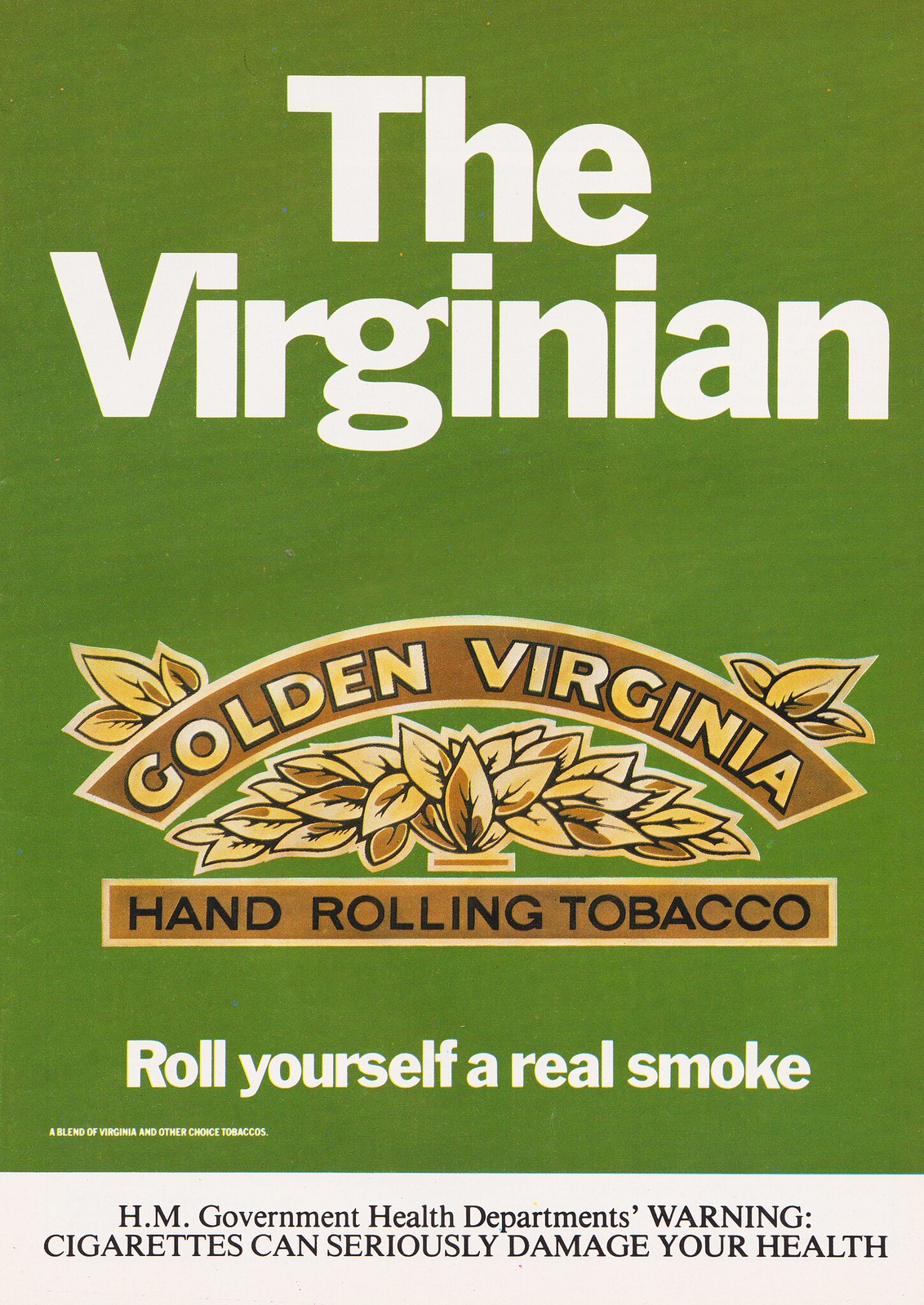The image depicts an advertisement from an older magazine featuring a rectangular, vertically-oriented front of a pack of cigarettes with a predominantly olive green background. At the top of the advertisement, in bold white text, is the brand name "The Virginian." Below this, there's a gold-colored semicircular logo with the text "Golden Virginia" on a light brown background, accompanied by an illustration of golden tobacco leaves spreading out from the center and corners of the arch. Directly below the logo, within a brown rectangular banner, the words "Hand-Rolling Tobacco" are printed in black text. Further down, in white bold letters, the tagline "Roll Yourself a Real Smoke" is prominently displayed, followed by the subtext in smaller white print stating, "A blend of Virginia and other choice tobaccos." At the very bottom of the page, a white banner features a health warning in black text that reads "H.M. Government Health Department's Warning: Cigarettes can seriously damage your health." The overall style and elements suggest a vintage advertisement for hand-rolling tobacco called "Golden Virginia."